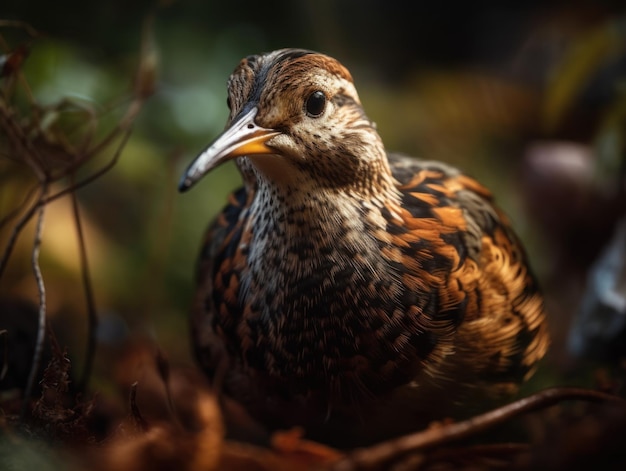The image showcases a woodcock bird, facing slightly to the left of the picture. The bird features primarily brown coloration with distinct markings and a notably long, sharp beak. Its head is brown with a defining black vertical stripe extending from the top of the head down towards the beak, which is segmented into a dark gray top, with white and orange hues at the bottom. The area around the eye is cream-colored below and tan brown above, with a dark gray line extending behind the eye. The bird’s wings display a rich blend of chestnut brown, black, and gray feathering, while the chest features a speckling of gray and black. The bird stands on a ground scattered with some twigs and branches, with additional branches visible on the left side. The background is generally dark and blurred, presenting shades of brown and green.